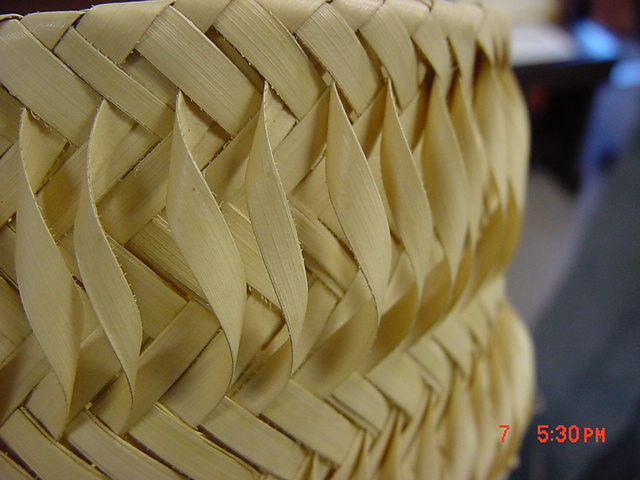The image depicts a well-crafted, interwoven structure made from a material that resembles either straw or bamboo, likely a natural palm or similar fiber. This structure features a distinctive tannish color, akin to the palm fronds used on Palm Sunday. The intricate weave dominates almost the entire image, with sharp clarity on the left side and becoming increasingly blurry towards the right. In the bottom right corner, there is a timestamp reading "5:30 PM" displayed in red numbers with a noticeable space between "5" and "30." Although the background is mostly obscured and blurry, faint shades of gray, white, brown, and a hint of blue are visible in the top right area of the image. The image could be representing a portion of a basket, possibly a large one, or even a piece of furniture like the side of a loveseat or couch, given the large size and skilled craftsmanship of the weave.